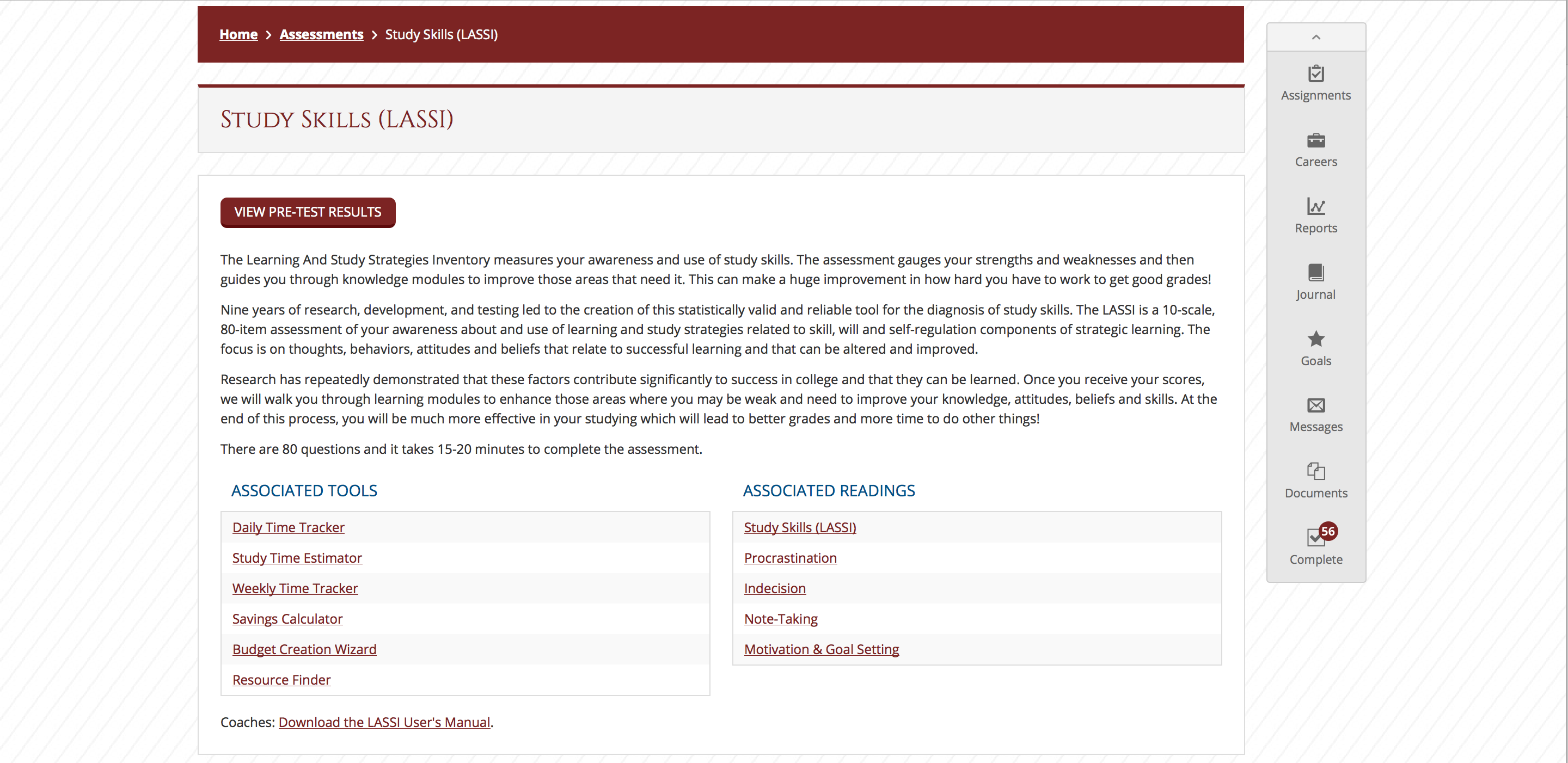The screenshot depicts a webpage dedicated to study skills, specifically focusing on the Learning and Study Strategies Inventory (LASSI). At the top of the page, a garnet-colored navigation bar with white text includes links labeled "Home," "Assessments and Study Skills," and "LASSI." The title of the page, prominently displayed, reads "Study Skills: LASSI." 

There is a button labeled "View Pre-Test Results" situated just beneath the title. The next section provides an overview of LASSI, detailing that it stands for Learning and Study Strategies Inventory. The LASSI is described as a tool developed through nine years of research, offering a statistically valid and reliable way to diagnose study skills. It is an assessment consisting of 80 items across 10 different skills, focusing on evaluating a person's awareness and use of learning and study strategies. The LASSI addresses components of skill and will, as well as self-regulation, targeting thoughts, behaviors, attitudes, and beliefs that contribute to successful learning and can be modified for improvement. 

Additional information highlights that the assessment comprises 80 questions and typically takes 15 to 20 minutes to complete. On the bottom left of the page, there is a section titled "Associated Tools" in blue, accompanied by garnet text links to features such as the Daily Time Tracker, Study Time Estimator, Weekly Time Tracker, Savings Calculator, Budget Creation Wizard, and Resource Finder. 

On the right side, another section titled "Associated Readings" lists links related to various topics, including Study Skills, LASSI, Procrastination, Indecision, Note-Taking, Motivation, and Goal Setting. 

Finally, there is a button provided for coaches to download the LASSI User's Manual.